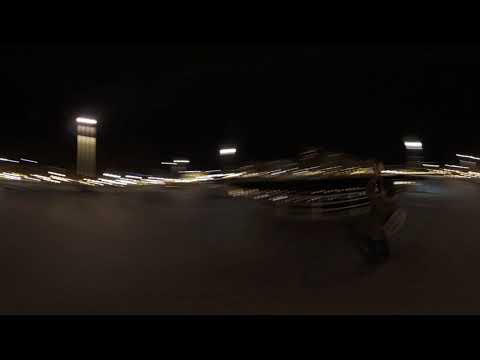The image, seemingly taken outside at night, reveals a dark upper section devoid of detail, transitioning to the middle where blurry white dots are scattered across. Dominating the left side is a tall, gray pillar with a distinct white stripe at its top, which contrasts with a shorter, rectangular object in the center and another similar structure to the right, both adorned with white stripes. The lower part of the image blends into a dark gray hue, indicative of pavement or open space, while the right middle section showcases an obscure, potentially moving figure amidst scattered white dots. Additionally, the scene features blurred city lights and glowing bars streaking across due to the motion during the photo capture. A faint outline of what could be a chair or cargo ramp is visible on the right, hinting at a possibly busy urban or airport backdrop.